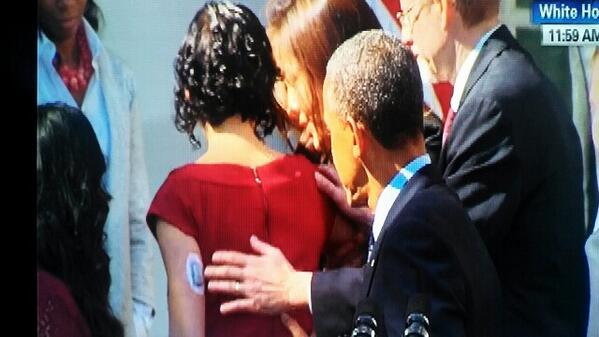This photograph features former President Barack Obama posing with a group of people. Among the group, a woman stands out in a striking red dress. On the back of her left arm, specifically in the tricep area, she has a circular white patch with a gray, bulging square component. The patch appears to be roughly three inches long and could potentially serve various medical purposes, such as an insulin monitor for diabetes management, a transdermal fentanyl patch, a bandage, or another type of medical patch.